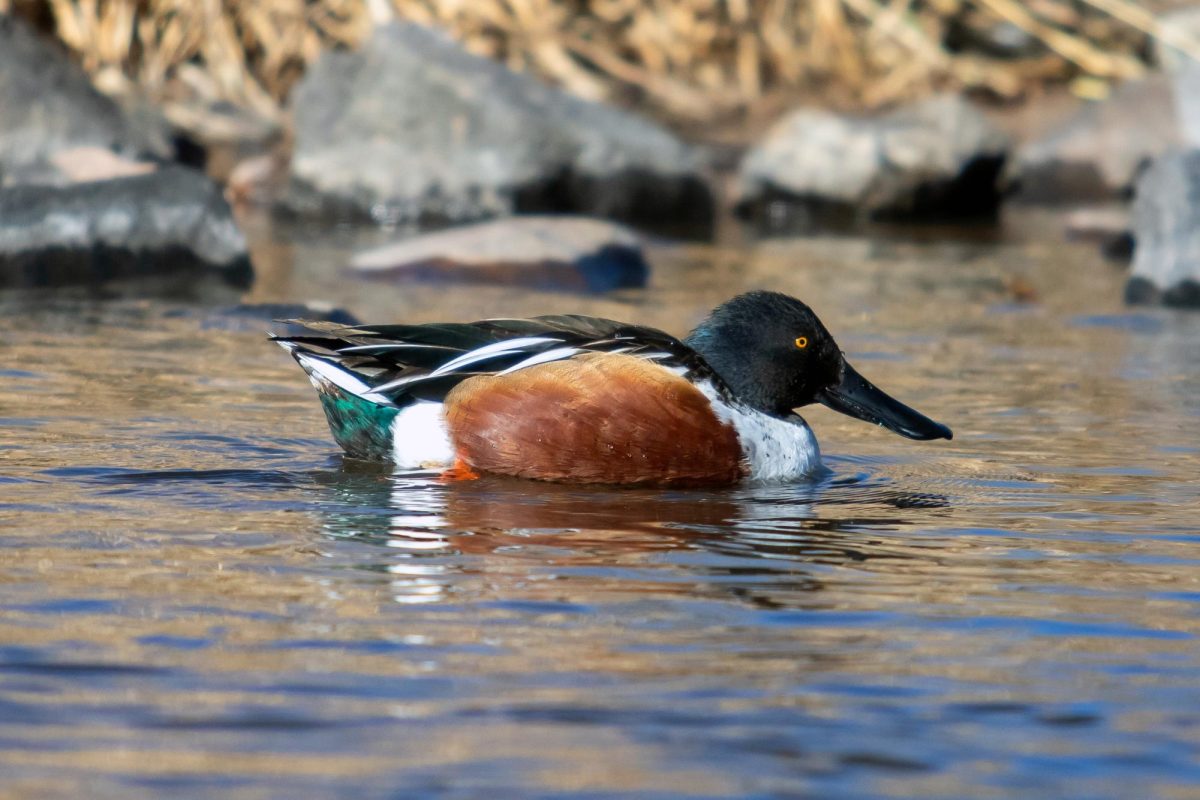This detailed photograph captures a mallard duck floating in dark blue water, paddling its orange feet. The duck is prominently positioned in the center of the image in crisp focus, while the background remains blurred. The background features gray boulders, rocks, twigs, and some brown grass or leaves, contributing shades of browns, grays, blues, and yellows to the scene. The mallard, shown in profile facing right, boasts a striking appearance with a black beak, black head, bright yellow eyes, a white chest, brown wings, and blue feathers on its back. The close-up reveals intricate details of the duck's plumage, with hints of green near its tail, making it a visually captivating and interesting subject amidst its natural outdoor habitat.